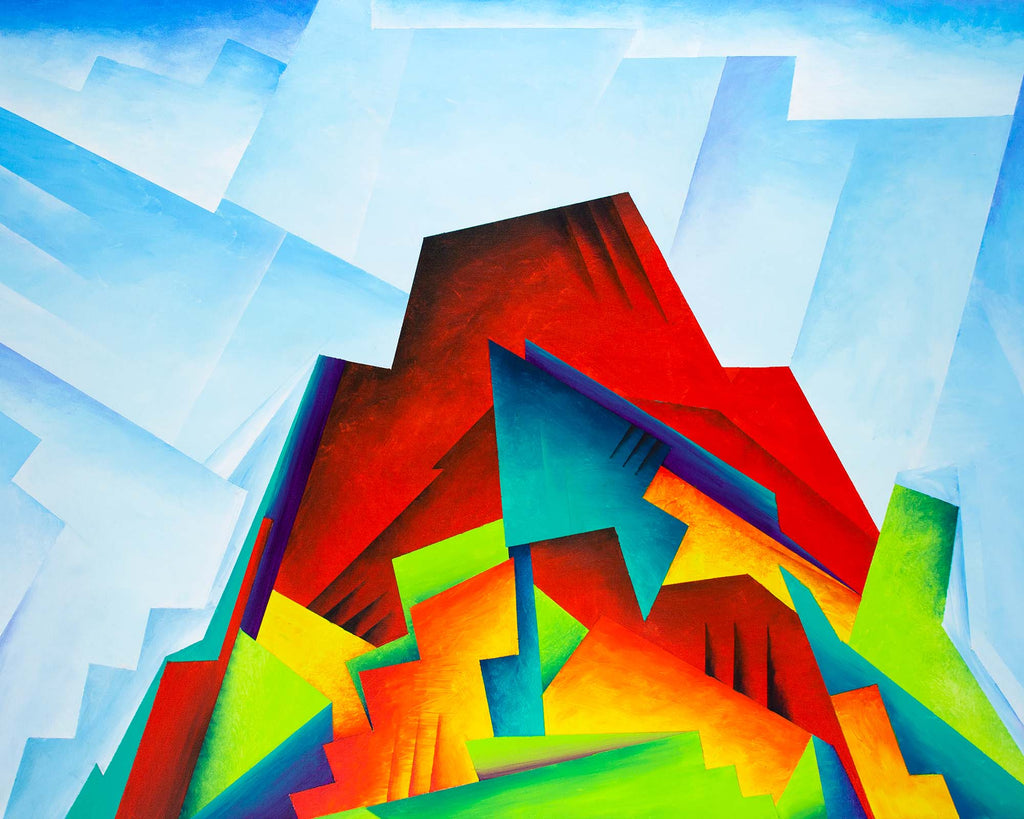This is an abstract painting of a mountain, characterized by its cubist style and bold, vivid colors. The mountain features a top peak in hot red shades with a black gradient surrounding the peak, creating an almost infrared effect. Below this, the mountain transitions into cooler tones like blue, green, yellow, and orange, with geometric divisions clearly marking the color changes. The formation is highly angular with a mix of squares, triangles, and rectangles, giving the mountain a sharp, jagged appearance.

The painting’s background depicts a sky composed of slanted geometric squares, transitioning in a gradient from darker blue at the top to lighter blue at the bottom. These shapes, like the mountain, are very squared off with no rounded lines, enhancing the overall geometric and angular aesthetic. The colors and shapes of the mountain pieces appear almost like a jumbled stack or puzzle, creating an abstract yet recognizable mountainous form. The harsh, clearly defined lines contribute to the painting’s distinctly cubist and geometric style.